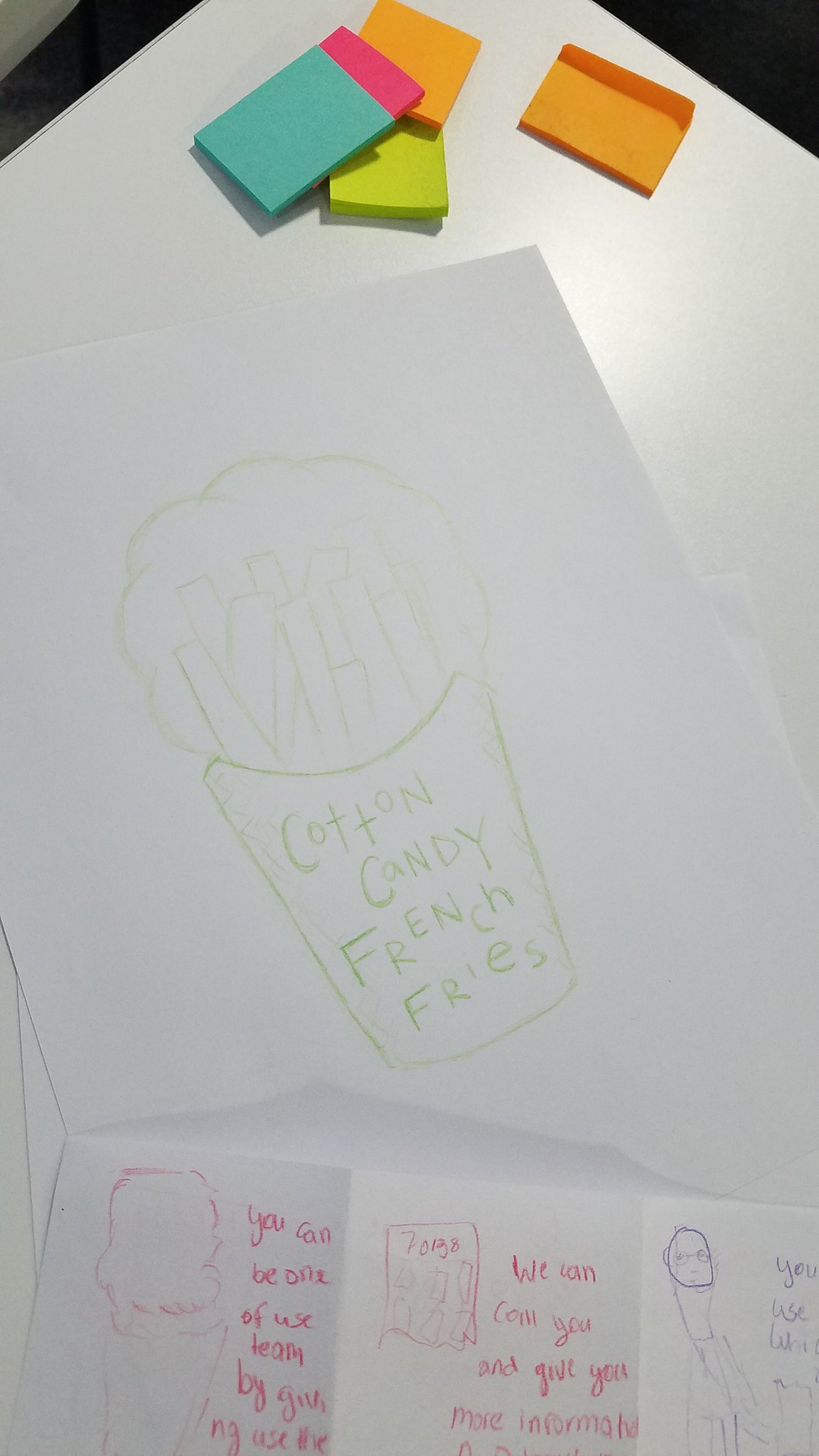The photograph captures a variety of drawings scattered across a shiny white desk. In the top portion of the image, the corner of the desk is cut off, revealing five small stacks of sticky notes in an array of colors: two orange, one lime green, one dark pink, and one blue. Dominating the composition is a large white sheet of paper featuring a detailed green pencil drawing of a box shaped like a container of french fries, labeled "Cotton Candy French Fries." The box design is clear, depicting fluffy clouds suggestive of cotton candy around the fries. In the foreground, there are additional folded sheets of paper adorned with indistinct drawings and handwritten notes in pink and purple. The scene presents a creative and colorful workspace.